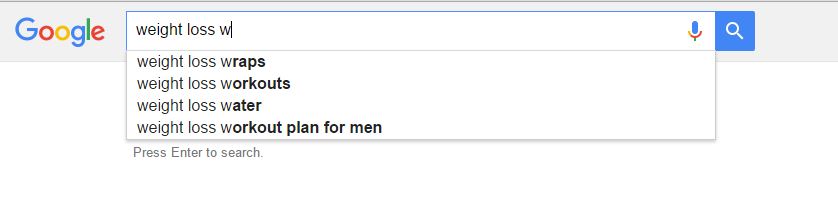The image displays a Google search bar, captured in landscape orientation, likely on a computer screen. At the top, a gray line is visible, followed by a prominent gray bar with the Google logo in vibrant colors: a blue 'G', a red 'O', a yellow 'O', another blue 'G', a green 'L', and a red 'E'. To the right of the logo is the search bar, accompanied by a microphone icon on its right side for voice search functionality, and the iconic search magnifying glass adjacent to it.

The search bar contains the partially typed query "weight loss W", triggering a dropdown menu below it that offers several suggested searches: "weight loss wraps", "weight loss workouts", "weight loss water", and "weight loss workout plan for men". Each suggestion is a clickable option that users can select to quickly refine their search. Above the suggestions, there's an indication to "press enter to search," allowing users to either choose one of the provided options or continue typing their own query. The dropdown list provides a convenient way to explore various weight loss-related topics beginning with 'W', enhancing the search experience.